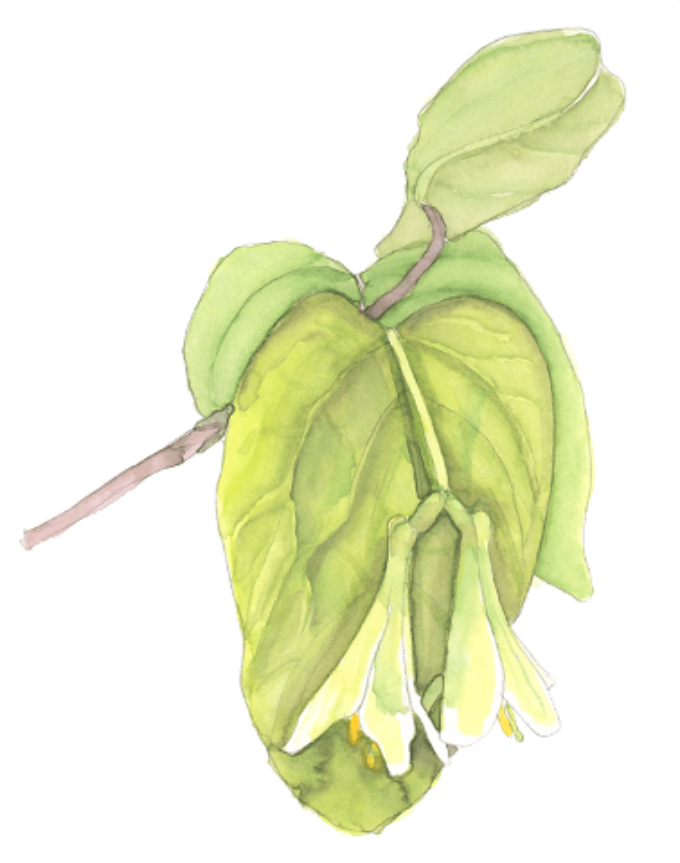The image presents a detailed watercolor painting set against a plain white background, with apparent dimensions of approximately four to five inches in height and three to four inches in width. At the focal point of the painting, a thin brown stalk begins just below the center on the left-hand side and ascends upward toward the upper right. This stalk is intersected by a prominent, long elliptical green leaf, which displays a yellowish hue and elongated heart shape with rounded tops and tapered ends. The leaf veins are rendered in a light greenish-gray tone.

Additionally, there is another green leaf positioned behind and slightly above the first leaf. Extending from near the base of the main green leaf, a thinner yellow stem branches out, splitting into two thicker stems from which two bell-shaped flowers hang downward. These flowers, appearing closed and not fully opened, exhibit a yellowish-green coloration with white-tipped petals and yellow stems. Overall, the leaves and flowers convey a soft gradient of light to possibly darker greens, enhancing the delicate, naturalistic quality of this botanical composition.